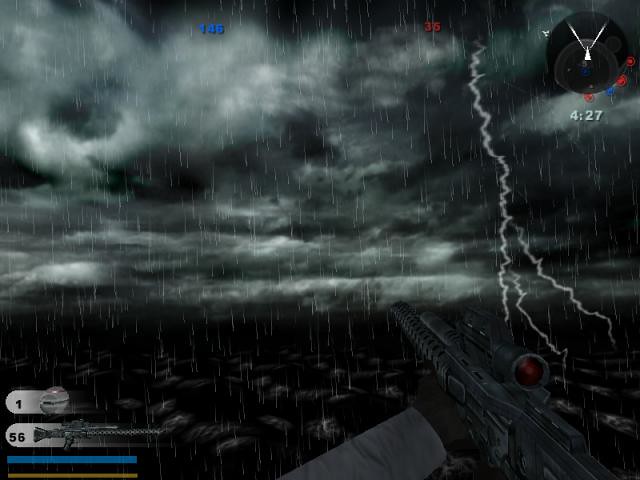In this color photo, the scene is shrouded in darkness, suggesting it is nighttime. The image portrays a violent storm with ominous clouds covering approximately two-thirds of the picture. The most striking element is a vivid lightning strike on the right side, which illuminates the tempestuous sky. The rainfall, rendered in white, cascades heavily, adding to the overall tumultuous atmosphere.

Below the horizon line, shrouded in the dark foreground on the right side, there is a silhouette of a gun, with a red sight, and a hand appears to be holding it. This suggests the player is in the first-person perspective of a video game. The left side of the image features a status display, possibly showing game statistics like weapon usage or player score, indicated by the number "56". Additionally, the top right corner of the image displays a timer reading "4:27" alongside other game-related indicators in red and blue.

The combination of these elements – the storm, the lightning, the rain, the gun, and the game interface – creates an intense and immersive scene from a video game.